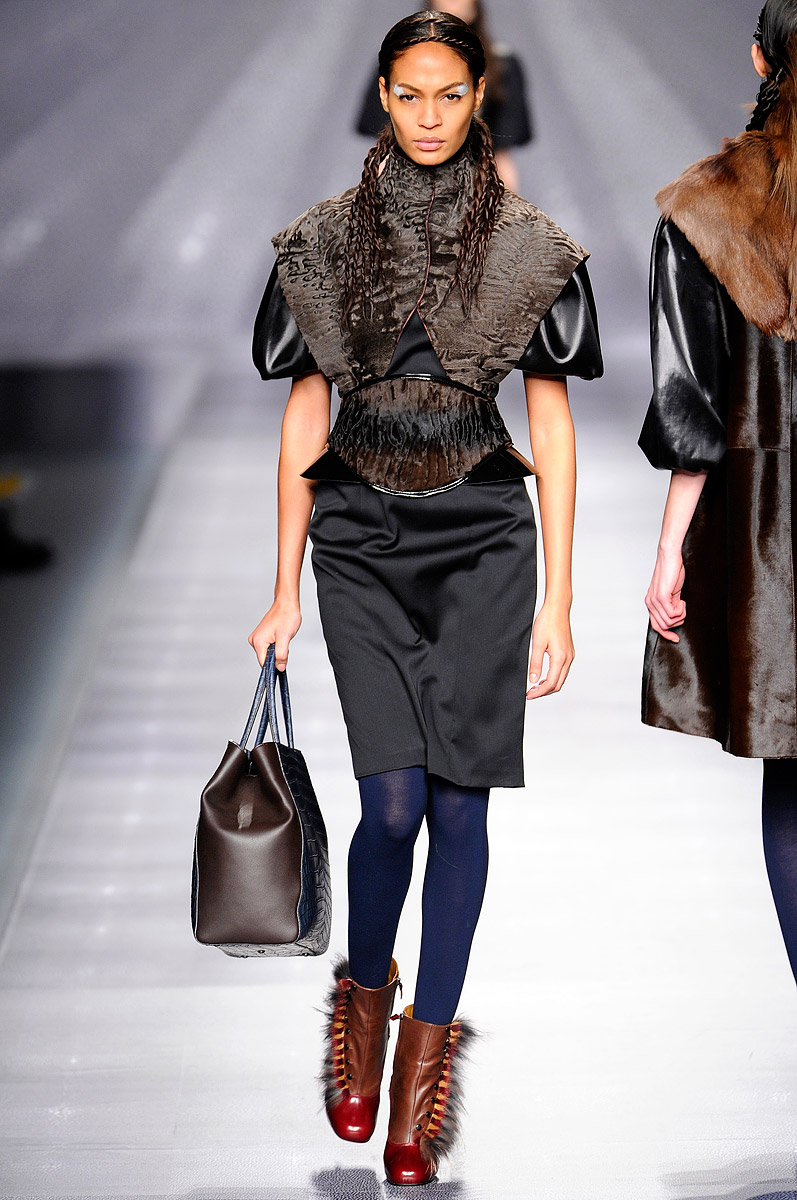The image captures a striking scene from a fashion runway show. At the center is an elegant African American female model, walking confidently towards the camera. Her outfit is a stunning blend of textures and colors: she's donned in a high-neck, shimmery dark brown vest paired with a voluminous black dress that features large sleeves. Below, she wears distinctive blue leggings and unique brown, feathery boots that reach just below her calves. Her hair is intricately braided and falls gracefully in front of her, complementing her sophisticated look, enhanced by bold black eye makeup. In her hand, she carries a sleek black designer purse.

To her immediate left on the right side of the image, another model is visible, walking in the opposite direction, dressed in a black sweater with a large, fluffy brown collar. There is also a blurred figure of a third model behind the main subject, just starting her walk down the glossy, whitish-gray runway. The scene is bustling with high fashion energy, showcasing the thrilling dynamics of a live runway event.